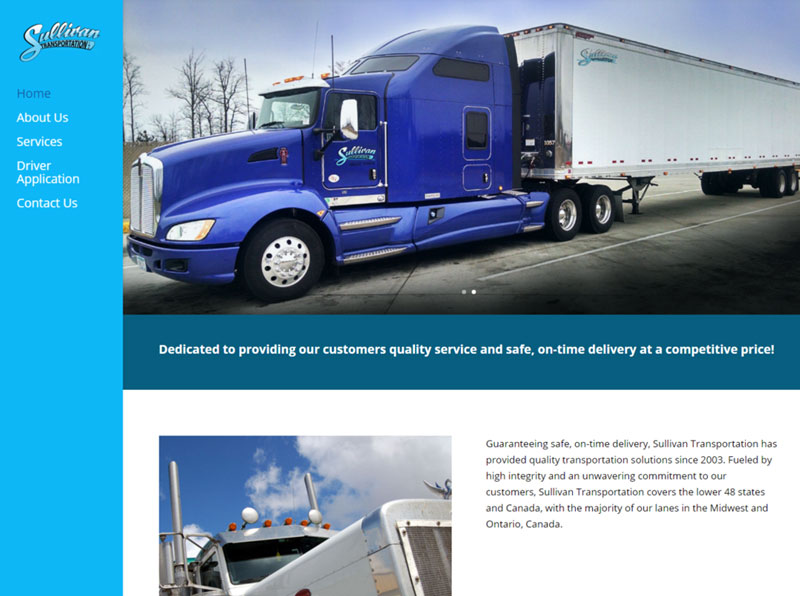The image features a website layout for "Sullivan Transportation." 

In the upper left corner, the logo reads "SULLIVAN Transportation." A vertical blue navigation bar on the left side contains white text for links labeled "Home," "About Us," "Services," "Driver Application," and "Contact Us," with "Home" highlighted in blue, indicating the current page.

Dominating the main content area is an image of a blue big rig truck with a sleeper cabin and a white trailer. Below this image is a slogan in dark teal color with white font that reads: "Dedicated to Providing Our Customers Quality Service and Safe On-Time Delivery at Competitive Prices."

Further down, another photo of a big rig truck shows just the engine and front window, overlaid with text that states: "Guaranteed Safe On-Time Delivery." Additionally, a paragraph explains Sullivan Transportation's history and services: "Since 2003, Sullivan Transportation has provided quality transportation solutions, fueled by high integrity and an unwavering commitment to our customers. Sullivan Transportation covers the lower 48 states and Canada, with the majority of our lanes in the Midwest and Ontario, Canada."

The color scheme of the site includes sky blue, royal blue, and teal blue accents.